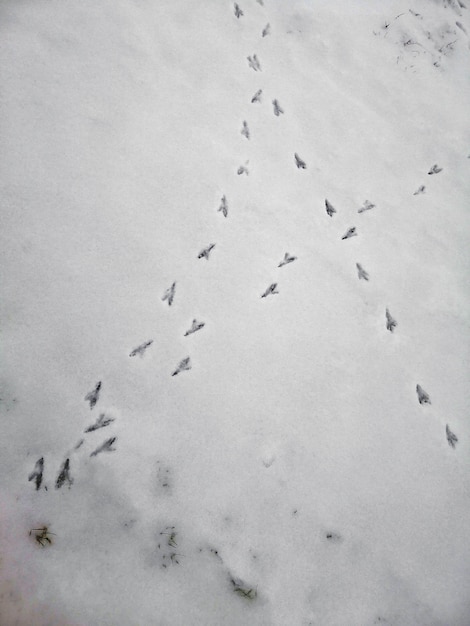This monochromatic photograph captures a stark, cold scene of thin, icy snow on the ground, with multiple sets of small bird tracks crisscrossing in various directions. The bird footprints, which appear dark against the white snow, form a pattern resembling the letter "A." One set of tracks starts from the lower left, arcs up to the top middle, while another set moves from the upper right towards the lower left, and yet another begins at the lower right and travels upward. Small patches of grass and tiny rocks poke through the snow, adding subtle details to the otherwise desolate, wintry landscape.